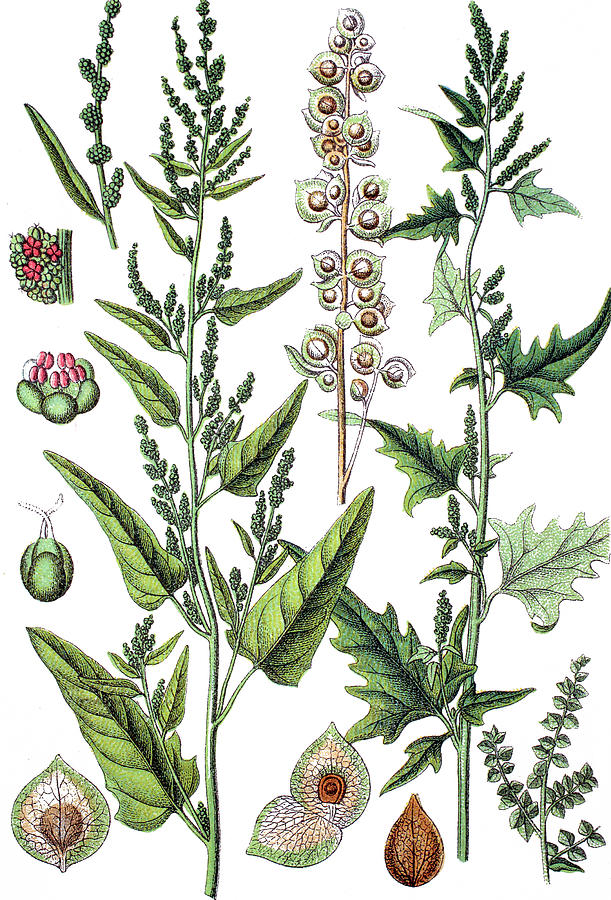This detailed illustration features various plants and their specific parts against a white background, reminiscent of botanical drawings from a turn-of-the-20th-century scientific book. The image comprises four distinct plant types displayed from left to right. Each plant is meticulously depicted, highlighting leaves, branches, and budding regions, with some areas shown in detailed close-ups.

On the left, there is a tall plant with a brown stalk, notable for its sinister-looking buds. Adjacent to it are leaves that resemble those of a cactus, extending into long, detailed stems. These leaves and stems vary in size and are intricately drawn, showcasing a range of shapes, from triangle-like structures to Christmas tree silhouettes.

The center features another tall plant with green leaves and eye-like buds, suggesting a grain or weed species. Here, the focus is on the fruiting bodies, which are devoid of flowers but rich in grain-like buds.

On the right, there is a darker-hued plant with similar buds, contrasting the predominantly green landscape. Scattered throughout the drawing are smaller plants and buds, adding to the diversity of the scene. A subtle splash of color is presented by occasional pink and slight red hues on some of the berries and leaves, contributing to the overall vibrant yet scholarly depiction of various flora.